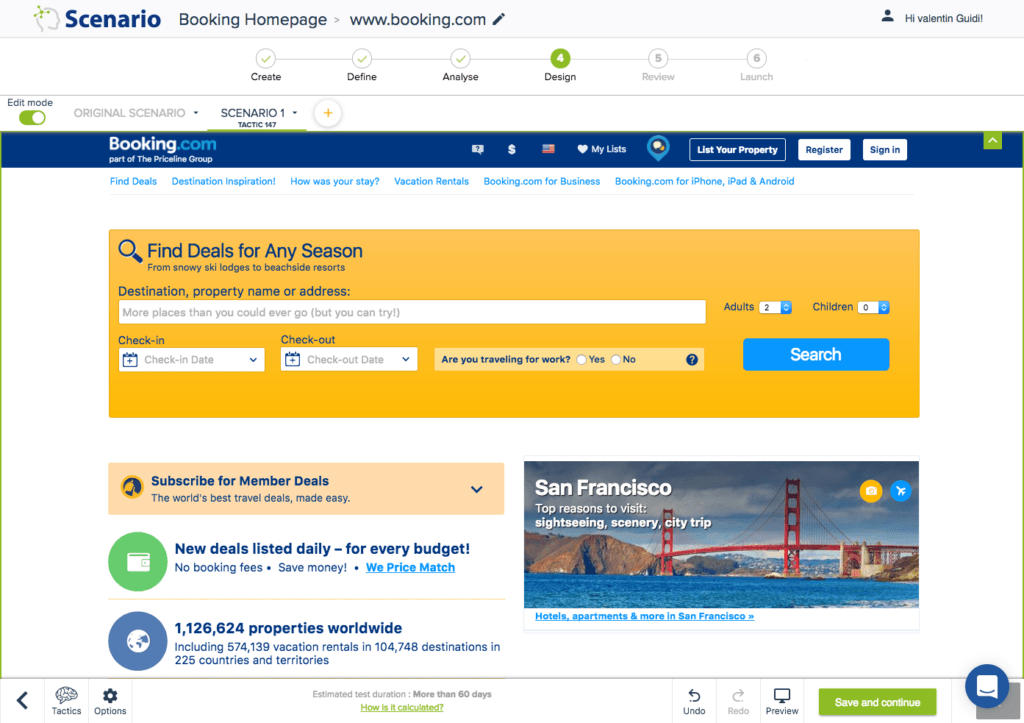Here is a cleaned-up and highly detailed caption for the image of the booking website:

---

This image captures the homepage of a booking website, specifically www.booking.com. In the top left, there's an icon resembling a human head or face, followed by the words "Scenario" in bold blue. The site URL www.booking.com is displayed next to this. The user profile displayed belongs to Valentin Guidi. The webpage is organized into six phases - Create, Define, Analyze, Design, Review, and Launch - and the current screen is on the 'Design' phase.

Below a line break, there is an 'Edit Mode' option. The screen highlights the original scenario labeled as "Scenario One" costing $47. Another line break follows, leading into the section header "www.booking.com: Part of the Priceline Group." Here, various icons are displayed, including a money icon, message icon, an American flag icon, a 'My List' heart icon, and a location icon. Options provided include "List Your Property," "Register," and "Sign In."

Beneath this, hyperlinks such as "Find Deals," "Destination Inspiration," "How Was Your Stay," "Vacation Rentals," "booking.com for Business," and "booking.com for iPhone, iPad, and Android" are listed. Below, a yellow rectangular box invites users to "Find Deals for Any Season from Snowy Ski Lodges to Beachside Resorts," allowing input for destination, property name, and address. Settings are pre-configured for two adults and zero children, with options to select check-in and check-out dates and to specify if traveling for work. A "Search" button facilitates information retrieval.

Further down, a smaller box prompts users to "Subscribe for Member Deals" with the tagline "The world's best travel deals made easy," and an arrow for more options. A bold statement below highlights "New deals listed daily for every budget. No booking fees. Save money. We price match." Specific metrics are provided, indicating 1,126,624 properties worldwide, including 574,139 vacation rentals, spanning 104,748 destinations across 225 countries and territories.

To the right, an image of the San Francisco Bridge with the caption "San Francisco" is shown. Top reasons to visit include sightseeing, scenery, and city trips, accompanied by camera and airplane icons. Below are hyperlinks featuring "Hotels," "Apartments," and more in San Francisco.

At the bottom of the screen, the footer contains buttons for "Tactics" or "Options." A message mentions an estimated test duration of more than 60 days with a clickable link "How is it calculated." Further right, options to "Undo," "Redo," "Preview," and "Save and Continue" are visible.

---